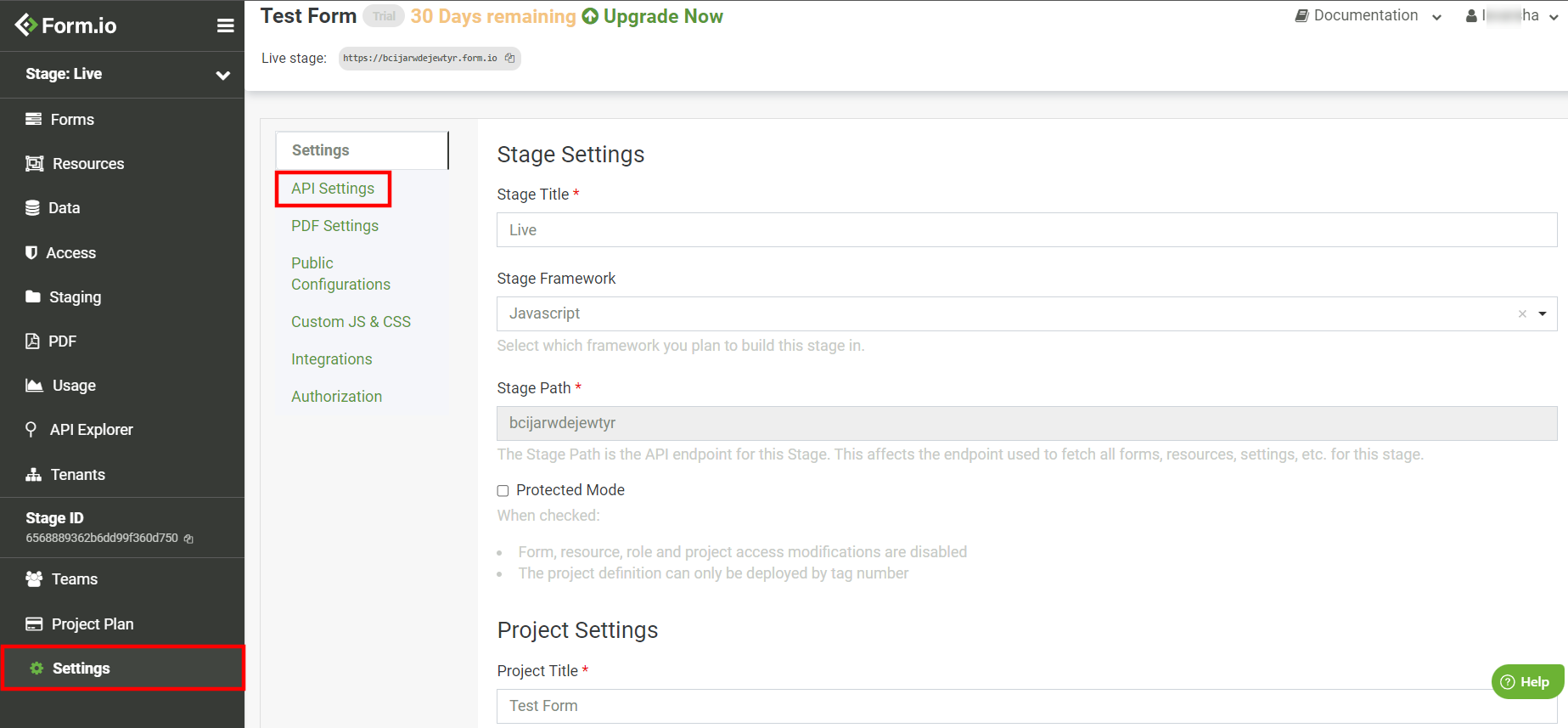This screenshot features a cropped view of a panel within the Form.io application. The left side of the image showcases a vertical black column adorned with the Form.io logo at the top left corner. Below the logo, an array of categories is listed, beginning with "Stage Live," which includes a drop-down menu situated to its right.

Continuing downward, the vertical list of categories includes: Forms, Resources, Data, Access, Staging, PDF, Usage, API, Explorer, Tenants, Stage ID, Terms, Project Plan, and Settings. The "Settings" category at the bottom is particularly emphasized with a red box superimposed around it.

To the right of this vertical column, a small panel labeled "Settings" is displayed with a white header. Below this header, several subcategories appear, starting with "API Settings," which is also marked by a red box for emphasis. To the right of this small panel, the main section of the image reveals the Stage Settings page.

Overall, this screenshot illustrates the sequence of navigating to "Settings," selecting "API Settings," and subsequently presenting the applicable Stage Settings page for further input and configuration.